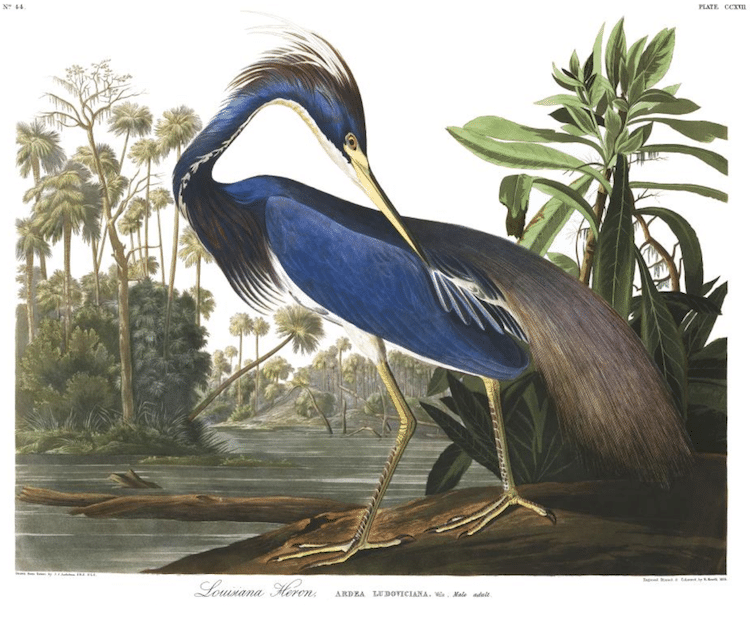This detailed illustration, titled "Louisiana Heron," showcases a striking blue bird set against a white background. The heron, with its long yellow beak and gold-colored, long legs, stands on the brown dirt of a riverbank. Its feathers are a harmonious blend of blue, gray, and black, with a distinguished brown and white top notch on its head. The bird's body is mostly blue, transitioning to lighter shades under its neck, and it gracefully turns its head to the right, displaying a poised stance with its beak above its back legs. Surrounding the heron, the scene is rich with nature: to the far left stands a tall tree, while the right side is dominated by lush green leaves of a large plant. The backdrop features a serene blue body of water, dotted with a horizontal log, framed by copious green trees that stretch into the horizon. This painting not only captures the elegance of the Louisiana Heron but also vividly brings to life its tranquil habitat.